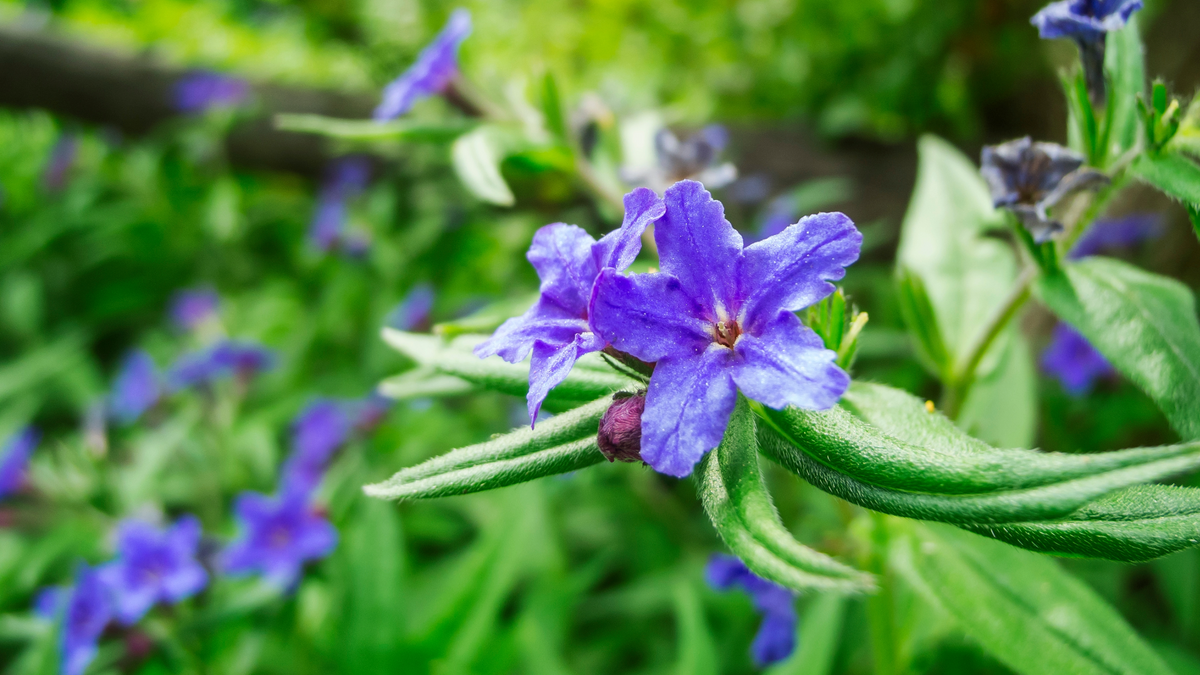The image showcases a stunning scene of purple flowers with five delicate petals, each adorned with lush green leaves. Prominently featured in the foreground is one sharply-focused flower, displaying its vibrant, velvety texture. Flanking it are two smaller blossoms and a single wilted bud, their stages of life highlighted artfully. In the background, the scene is harmoniously repeated with additional purple flowers and green foliage, subtly blurred to emphasize the central bloom. A faint brown tree branch is discernible, running horizontally behind the flowers, further enhancing the depth of the composition. Notably, on one of the front leaves, a small yellow dot—perhaps pollen—adds an intriguing detail, and the leaves exhibit a soft, fuzzy texture that hints at their tactile nature. This intricate interplay of colors and textures creates a captivating botanical tableau.